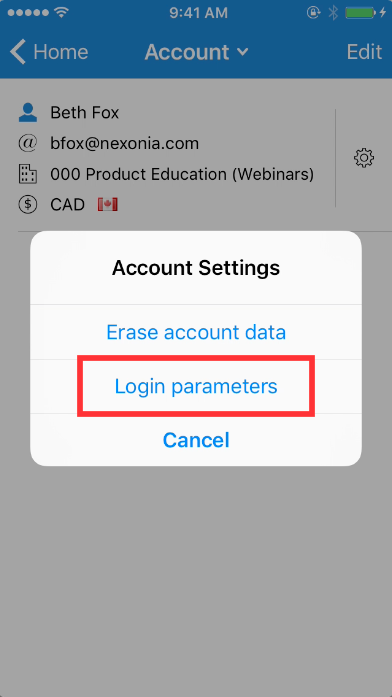This detailed caption describes a cropped screenshot of an account screen on a mobile phone app:

At the top of the screen, the word "Account" is prominently displayed in large white letters, centered. To the left of the word "Account," an arrow pointing to the left is labeled "Home" in white letters. Adjacent to the right of the word "Account," there is a small drop-down box, and to the far right, the word "Edit" appears in large white letters.

The area below these elements features a white background. At the top of this section, a profile icon is displayed with the name "Beth Fox" written to its right. Directly below the name, there is an "at" symbol followed by an email address. Under the email, a building icon indicates the person’s career information, which is listed beside it. Beneath these details, there is a dollar sign followed by "CAD" and a small Canadian flag.

In the center of the screen, a pop-up box appears, with the phrase "Account Settings" written at the top in large black font. Below this heading, there are three options: "Erase Account Data," "Login Parameters," and "Cancel." The option "Login Parameters" is highlighted with a red box edited into the photo to draw special attention to it.